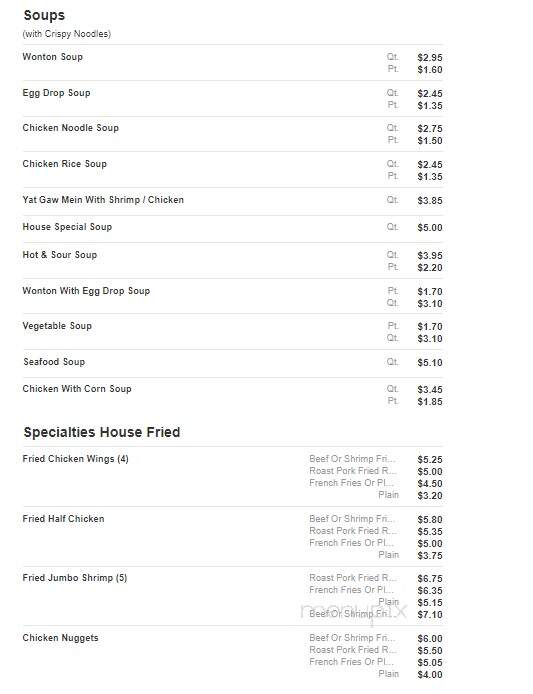Screenshot of Website Menu:

The screenshot captures a detailed view of a website menu, positioned vertically on the top left-hand side of the webpage. The background is predominantly white, providing a clear and clean display of the menu items.

**Soups:**
- **Crispy Noodles:**
  - **Wonton Soup:** 
    - Quart: $2.95, Pint: $1.60
  - **Egg Drop Soup:** 
    - Quart: $2.45, Pint: $1.35
  - **Chicken Noodle Soup:** 
    - Quart: $2.75, Pint: $1.50
  - **Chicken Rice Soup:** 
    - Quart: $2.45, Pint: $1.35
  - **Yat Go Mein with Shrimp/Chicken:** 
    - Quart: $3.85
  - **House Special Soup:** 
    - Quart: $5.00
  - **Hot and Sour Soup:** 
    - Quart: $3.95, Pint: $2.20
  - **Wonton with Egg Drop Soup:** 
    - Quart: $3.10, Pint: $1.70
  - **Vegetable Soup:** 
    - Quart: $3.10, Pint: $1.70
  - **Seafood Soup:** 
    - Quart: $5.10
  - **Chicken with Corn Soup:** 
    - Quart: $3.45, Pint: $1.85

**Specialty House Fried:**
- **Fried Chicken Wings:**
  - Beef or Shrimp: $5.25
  - Roast Pork: $5.00
  - French Fries or Plain: $4.50, $3.20
- **Fried Half Chicken:** 
  - $5.80, $5.35, $5.75
- **Fried Jumbo Shrimp:** 
  - $6.75, $6.35, $5.15, $7.10
- **Chicken Nuggets:**
  - $6.00, $5.50, $5.05, Plain: $4.00